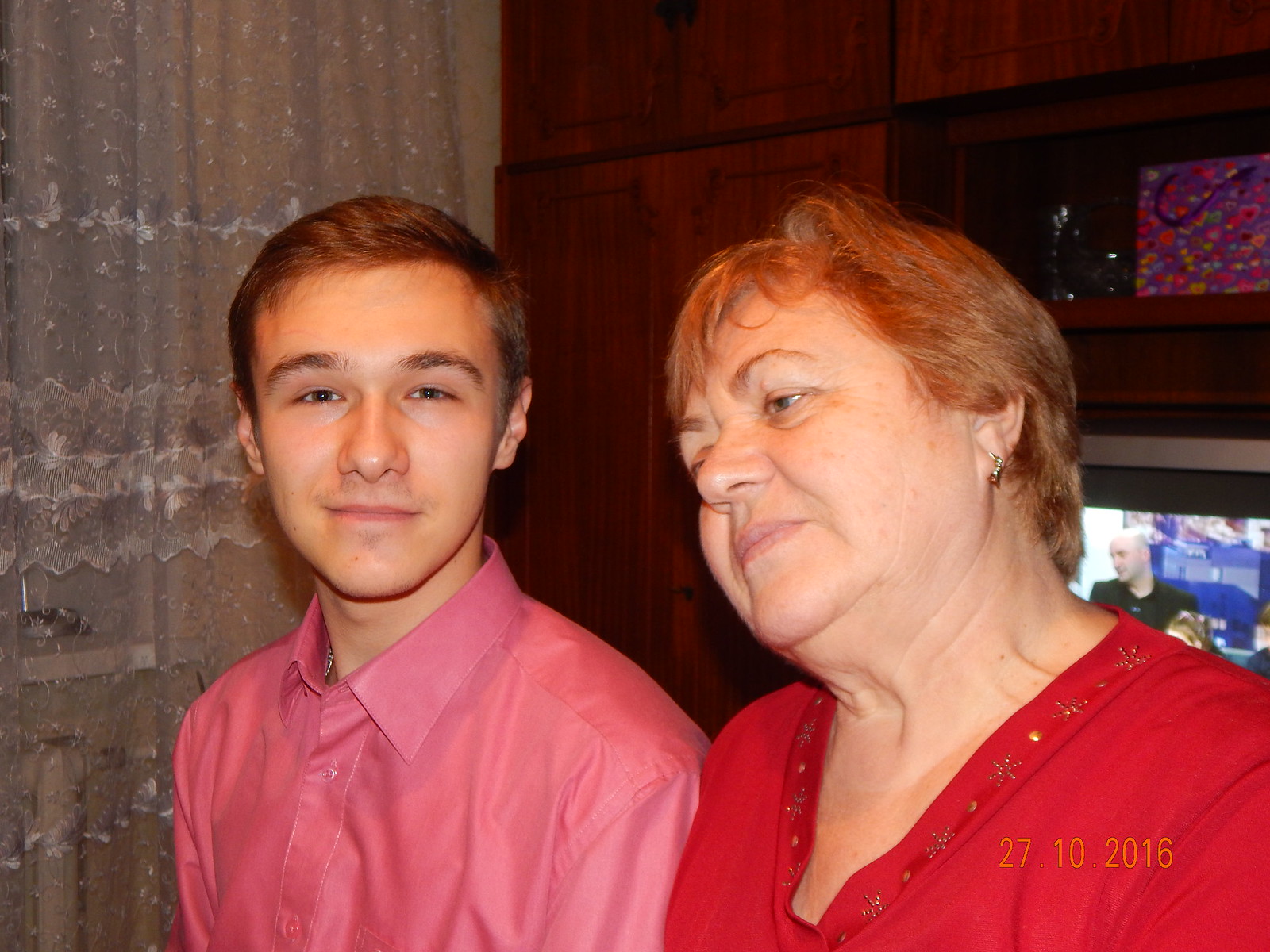In this well-lit indoor setting, two people are captured posing together. On the left, a young man with short brown hair and fair skin is dressed in a pink button-up shirt, revealing a small bit of a necklace underneath. He sports a slight smile and is looking directly into the camera. To his right, an older woman with short light brown hair, graying slightly, is seated. She is wearing a red v-neck blouse adorned with intricate gold embroidery along the neckline and small earrings. She tilts her head to her left, her expression suggesting she’s examining something. Behind them, white lacy curtains with floral designs are visible to the left, while a dark wooden panel console extends up to the ceiling on the right. Part of a TV screen displaying a scene, possibly a sermon, is also visible in the background. Together, they create a cozy and intimate scene with elements of a lived-in space around them.